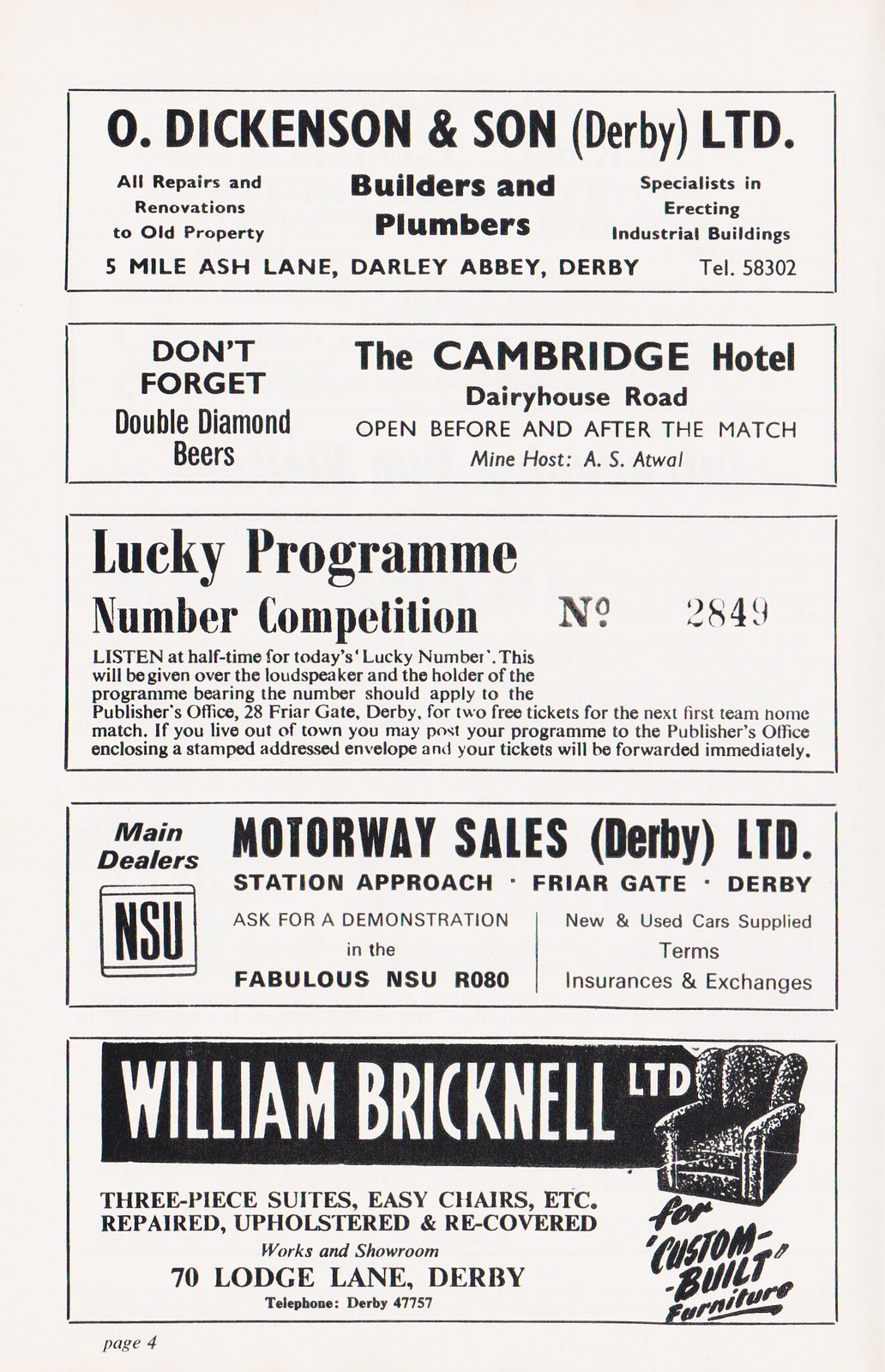The image displays a vertical white promotional flyer featuring five horizontally aligned advertisements, each outlined in black rectangles. 

At the top, the first ad prominently displays "O. Dickinson & Son Derby Ltd." with additional details such as "Builders and Plumbers," the address "Five Mile Ash Lane, Darley Abbey, Derby," and contact number "Telephone 58302." The services offered include repairs, renovations, and building specialists.

The second ad catches attention with the phrase "Don't Forget" and promotes "Double Diamond Beers." Adjacent to this, "The Cambridge Hotel" located on "Dairy House Road" is highlighted, followed by a few lines of additional text.

The third ad, on the upper left, reads "Lucky Program Number Competition" and under this are several lines of small black print. The details include an invitation to listen at halftime for the lucky number announced over the loudspeaker, with instructions for the holder of the winning number (2849) to visit the Publisher's Office at "28 Friar Gate, Derby" for two free tickets to the next first team home match.

The fourth ad features "Main Dealers Motorway Sales Limited" along the top, located at "Station Approach, Friar Gate, Derby." The services advertised include asking for demonstrations of the "Fabulous NSU R080" and mention of new and used cars being supplied, with insurance exchanges available.

The fifth and bottom ad stands out with a bold black background and large white text that reads "William Bricknell Ltd." An illustration of an easy chair is positioned below this text, to the right. The ad offers services for repairing, upholstering, and recovering furniture, including three-piece suites and easy chairs. The address given is "70 Dodge Lane, Derby," and the contact number is "Telephone Derby 47757," emphasizing the availability of custom-built furniture.